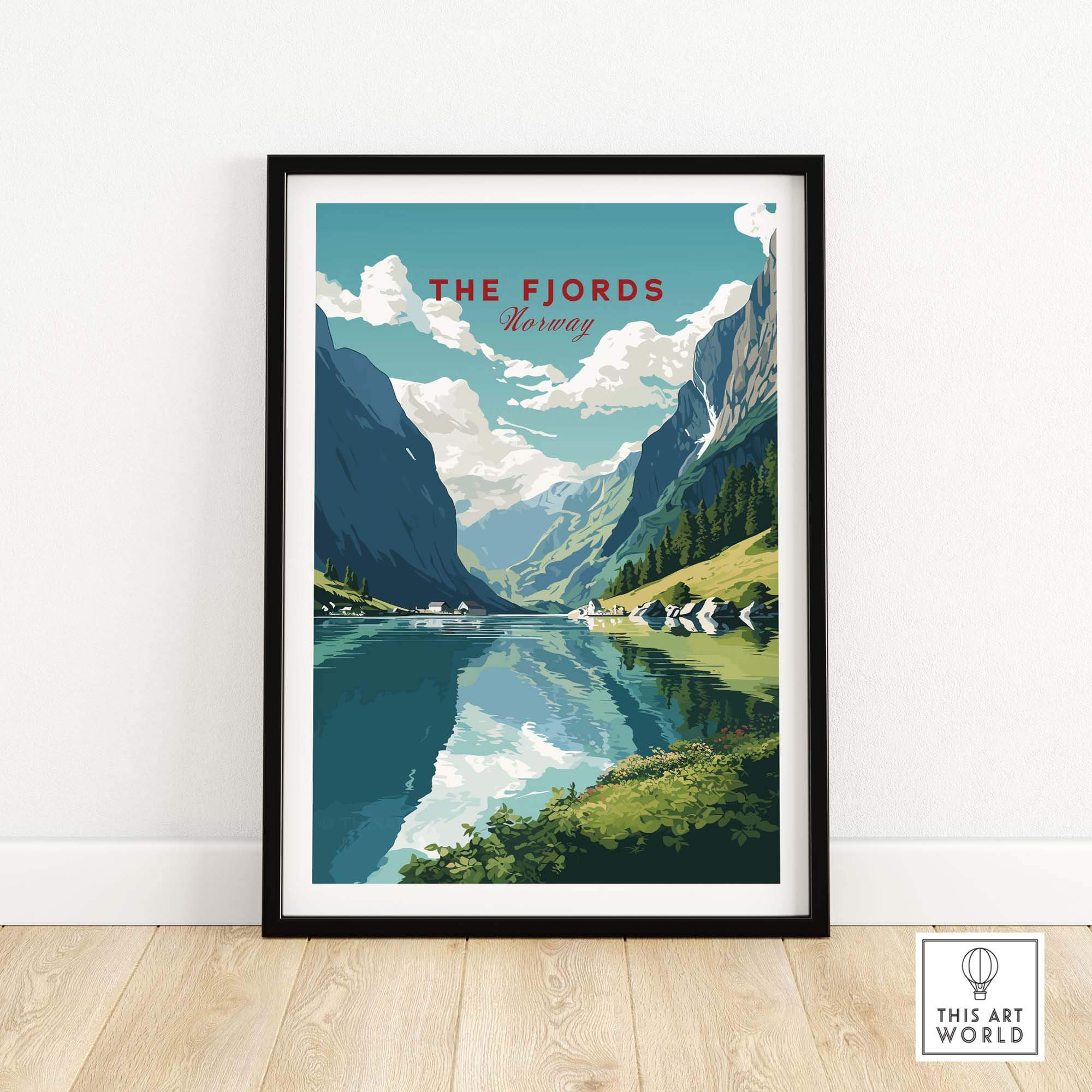This is a striking travel poster styled in a vintage fashion reminiscent of the era dominated by train travel advertisements. The large digital image, framed in an elegant black frame measuring approximately 22 by 26 inches, leans against a white wall above a light wood floor. At the top center of the poster, bold red text reads "The Fjords" with "Norway" elegantly scripted below in cursive, also in red. The background is adorned with towering mountains in shades of blue and green, under a sky painted light blue with scattered white clouds. The mid-ground features a serene body of water, mirroring the mountains and clouds in various hues of light green, white, and blue. Pine trees, green grass, and white rocks surround the water, giving a lush, natural feel. Nestled in the distance is a small house, adding a touch of human presence to the tranquil scene. In the foreground, vibrant green shrubbery and a cliff-like overlook enhance the picturesque composition. Notably, the bottom right corner of the artwork includes a small square with the text "This Art World" and an emblematic stick-figure hot air balloon, rounding off the artistic charm of this captivating portrayal of Norway's fjords.